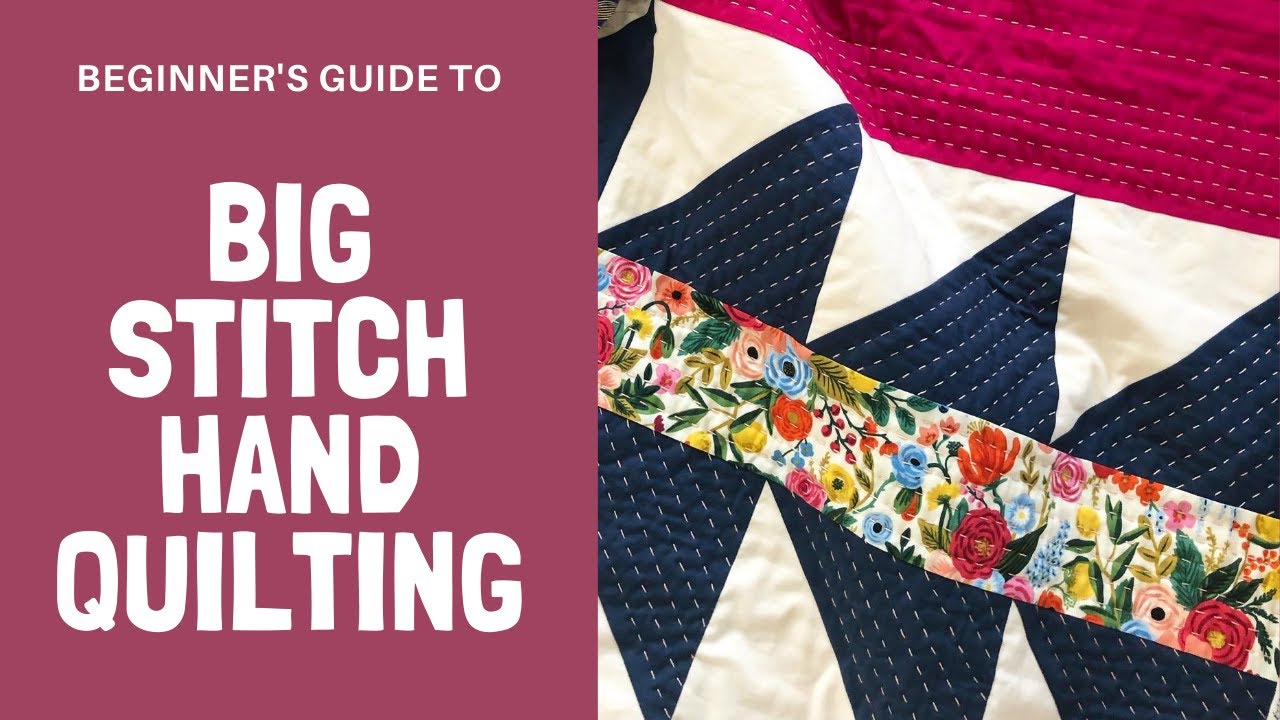The image features a probable book cover or online guide titled "Beginner's Guide to Big Stitch Hand Quilting." The left side showcases a maroon or plum-colored square with the title in white text; "Beginner's Guide to" is in a smaller font, while "Big Stitch Hand Quilting" stands out prominently in a large, easy to read font. The right side of the image displays a close-up of a quilt, emphasizing the hand-stitched details. The quilt portion includes a strip of red fabric at the top, followed by a broad section of white fabric that occupies the lower two-thirds of the image. On this white fabric, three navy blue triangles are arranged, with a continuous strip of colorful floral fabric—featuring orange, yellow, blue, pink, and red flowers, as well as leaves—running through the blue triangles. The visible irregular stitching highlights the hand-crafted nature of the quilt.